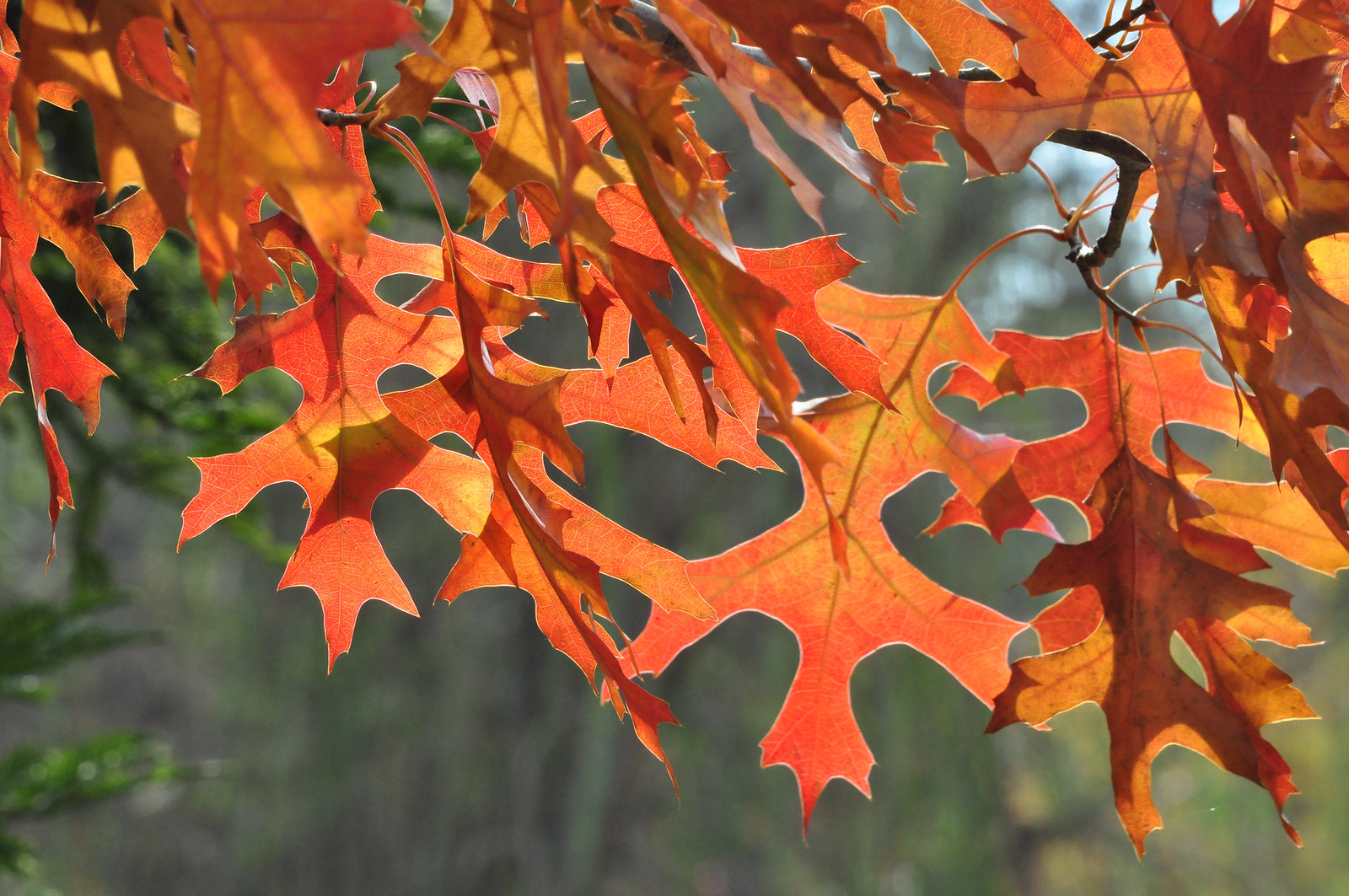A close-up image captures a cluster of large, elongated autumn leaves, which are a striking brownish-red hue. Each leaf features a prominent central vein, with three extended lobes on either side, creating a distinctive pattern. The leaves are tightly grouped together, partially supported by visible brown branches, though the tree they belong to remains out of sight. The perspective of the photograph is taken from below and slightly behind the leaves, providing a unique vantage point. In the background, a contrast is created by the vibrant green foliage of other trees, punctuated by patches of softer, blurred yellow tones. The sky, peeking through sporadically, reveals a clear, blue expanse, suggesting that the photo was taken during the daytime.